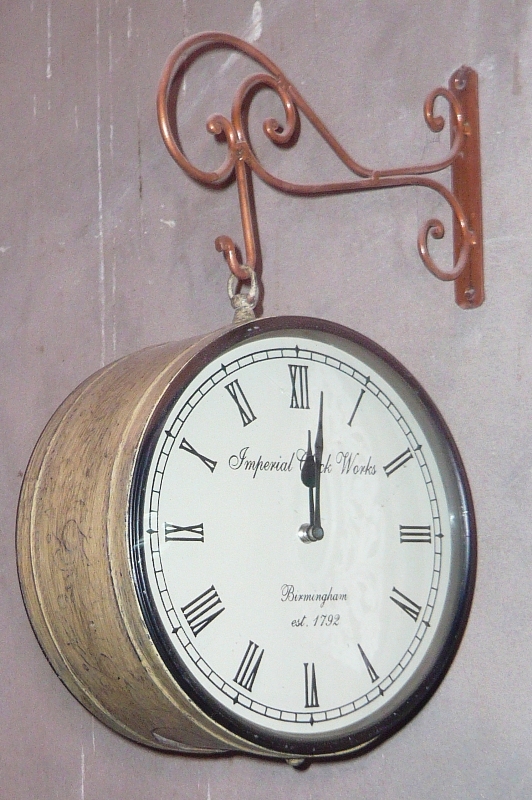This photograph captures a detailed view of an ornate, vintage-style clock hanging from a decorative copper-colored metal bracket, affixed to what appears to be a gray cement wall. The bracket is an intricate piece with spiral curls and loops, creating an aesthetically pleasing design. A small metal hook extends from the bracket, from which the clock is suspended by a silver ring. The clock itself is distinguished by its wide, barrel-like sides, resembling a deep encasement.

The face of the clock is white, adorned with black Roman numerals around its edge. At the top of the clock face, in cursive script, it reads "Imperial Clockworks." Below the hands, which indicate the time as two minutes past twelve, there is an inscription that reads "Birmingham, established 1792." The clock's wide, cylindrical body suggests that there might be an identical clock face on the opposite side, creating a double-sided timepiece. The color scheme features a mix of red and tan gray, contributing to its antique charm. The angle of the photograph provides a clear view of both the face and the intricately designed sides of the clock.